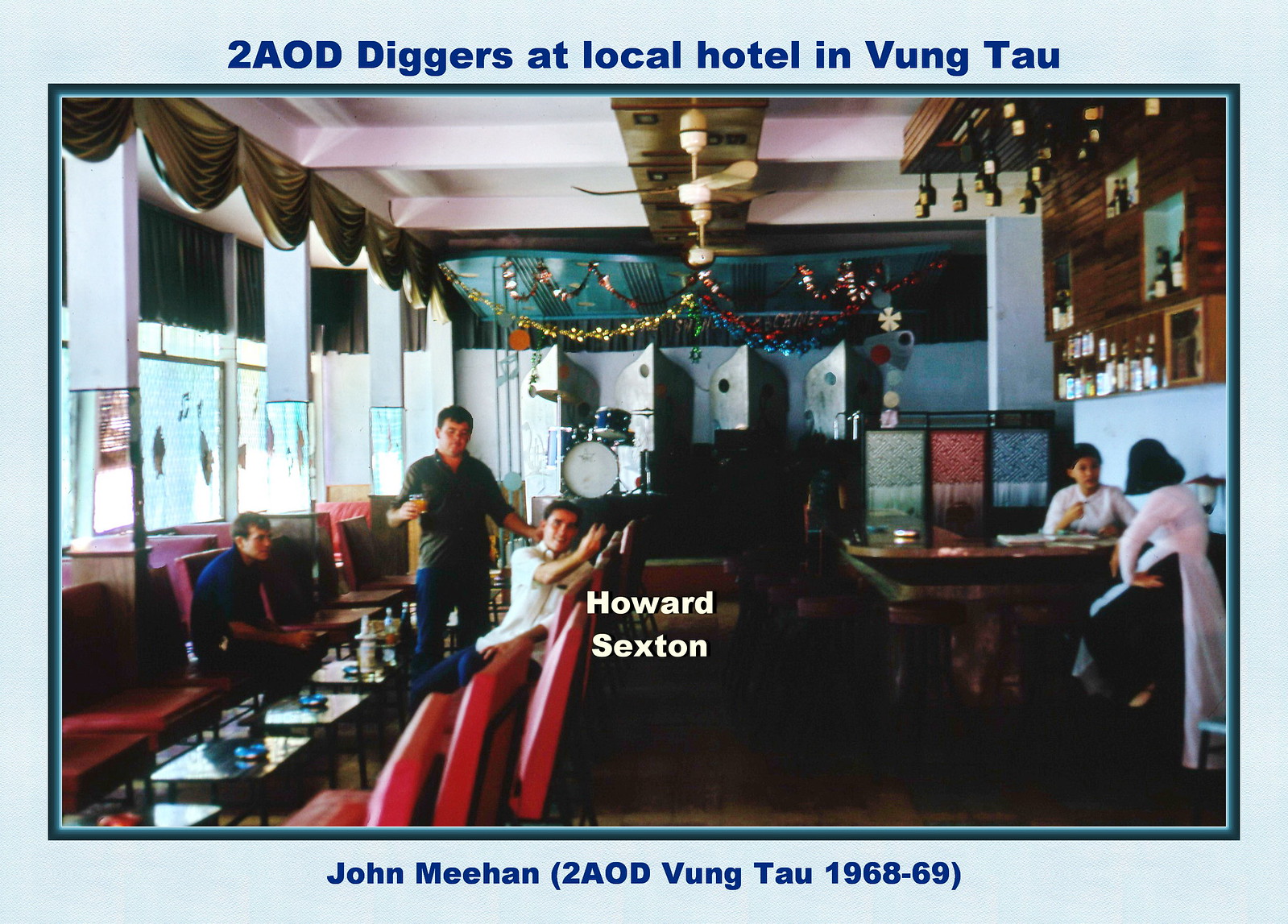This photograph from 1968-1969, taken in a local hotel or restaurant in Vung Tau, Vietnam, features three American men and two Vietnamese women. The backdrop includes wooden panels and red chairs, with hanging decorations and ceiling fans enhancing the ambiance. Two men are seated while one stands holding a drink, and the women are seen conversing at a table to the right. The image, evocative of the Vietnam War era, has text overlays identifying "Howard Sexton" and "John Meehan, 2 AOD, Vung Tau, 1968-1969." There is a stage with a drum set in the background, suggesting this could be a venue for leisure and gatherings, where the men might be reuniting and enjoying drinks.